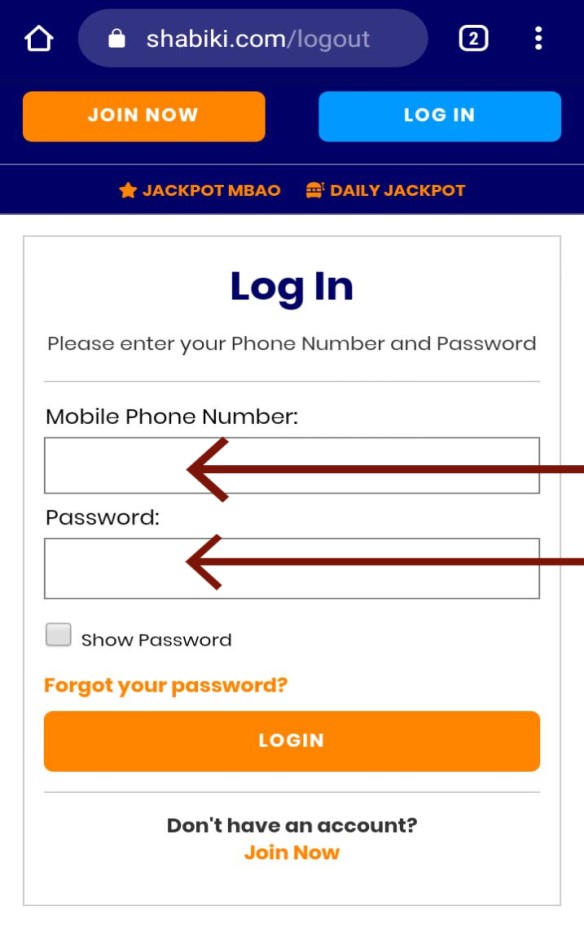Screenshot of an Android Device Webpage Displaying a Login Interface

This detailed screenshot depicts a webpage viewed on an Android phone. The URL in the browser at the top reveals the address "shahbaiqi.com/logout," indicating that the user is at the logout page of the site. On the top-right corner, there are two open tabs, while on the top left, a home key is positioned for easy navigation.

Beneath these elements, the primary focus turns to two prominent buttons. On the left side, an orange "Join Now" button is available, allowing new users to start the registration process. Conversely, on the right side, a blue "Login" button invites existing users to access their accounts.

Moving further down the screen, the main body showcases a login interface. Two dark red arrows draw attention to specific input fields; the first arrow points to a field where users can enter their mobile phone numbers, while the second arrow directs users to a field for entering their passwords.

At the bottom of the screen, an orange long "Login" button spans the width of the interface, facilitating account access. Above this button, a small link to the left reads "Forgot your password," providing a recovery option for users. Underneath the "Login" button, a caption reads, "Don't have an account? Join now," encouraging new users to sign up.